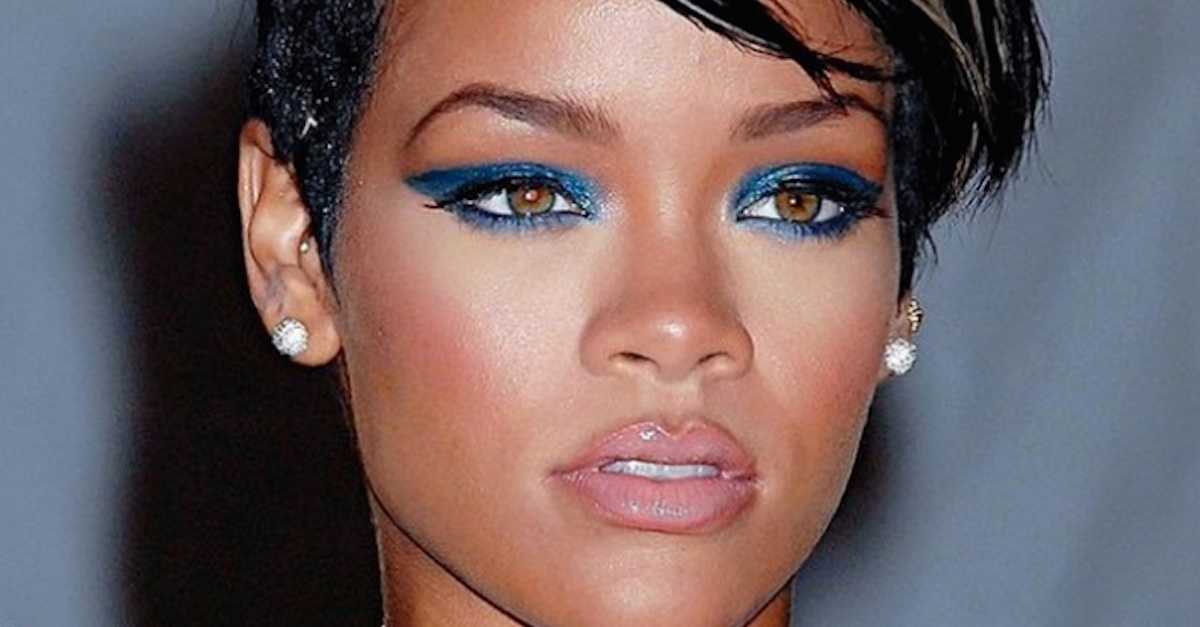This close-up photograph captures the face of singer Rihanna, with her forehead and chin partially out of frame. She is wearing a shimmering blue eyeshadow that surrounds her eyes, complemented by eyeliner and mascara for her long, black eyelashes. Rihanna's lips are colored with pink lipstick, and her short black hair frames her face, with her gaze directed slightly to the right. The photograph highlights her diamond-like round earrings in each ear against a gray background. Notably, the image appears somewhat pixelated with visible compression artifacts, suggesting it may have been cropped from a larger photo. A light shine is visible on the center of her face, likely from a flash used during the photography.